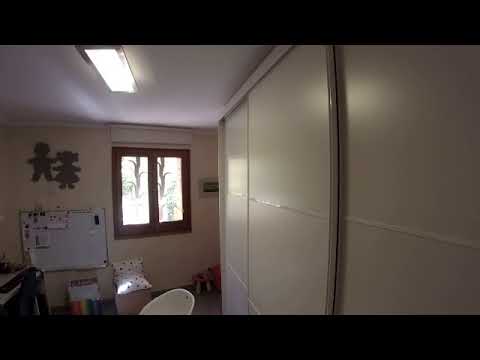The image captures the interior of a child's room, characterized by warm peach-colored walls and a bright, white ceiling with a rectangular light fixture. The window on the right, divided by brown bars into two rectangular panes, allows ample sunlight to flood the room. Beneath the window, there are cardboard cutouts of a brown-haired girl and boy, adding a whimsical touch to the space. On the left side of the room, a portion of a wooden framed object—possibly a crib or changing table—comes into view, partially obscured by a large black item resembling a puffy jacket. Scattered throughout the room are child-sized furnishings, including a small pink stool, white chair, and matching cushion. A whiteboard adorned with papers is fixed to the wall, further suggesting the room’s dual purpose as a playful yet functional children’s area.